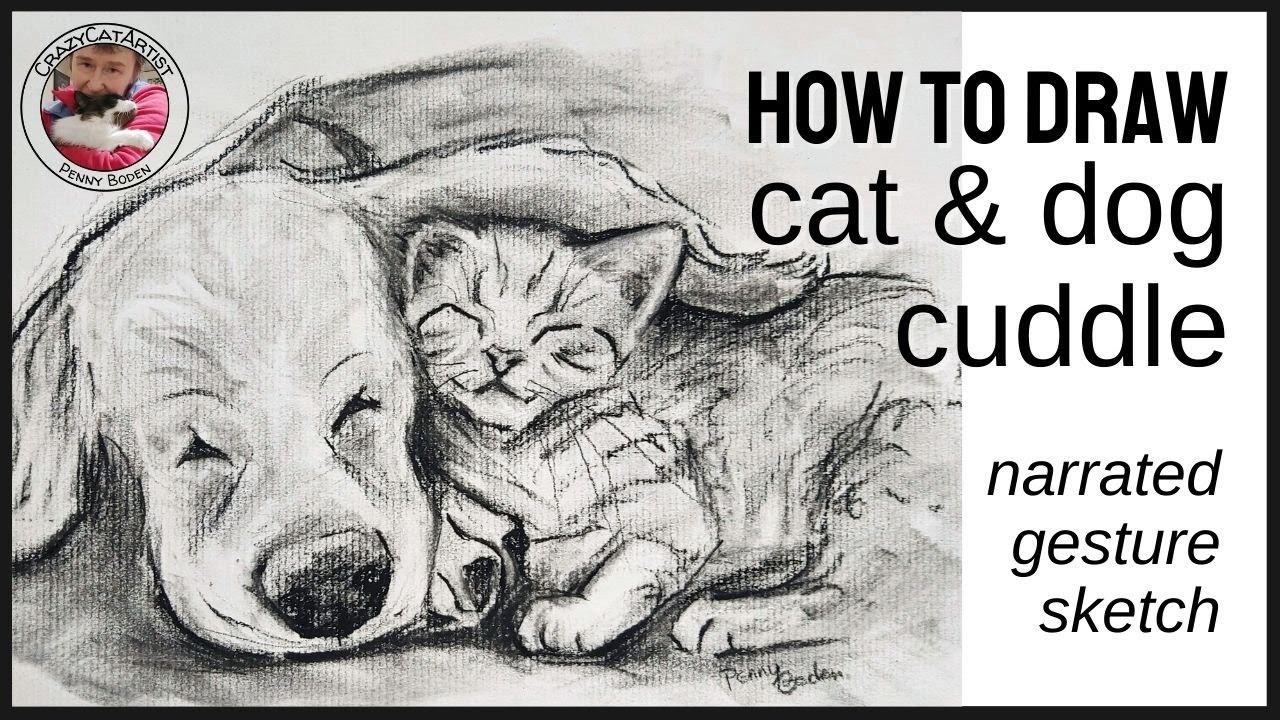The image is a vertically aligned rectangular sketch with a black border. Dominated by shades of brown and white, it is carefully penciled to depict a serene scene. On the left and middle sections, the drawing shows a dog resting with its head down and its eyes closed, while a cat cuddles next to it, nestled under the dog's floppy ear. Both animals appear tranquil and are drawn with fine detail, highlighting their closed eyes and content expressions.

In the upper left corner of the image, there is a circular emblem. This emblem contains a smaller image of a man holding a cat, with the text "Crazy Cat Artist" encircling it. Beneath this, the name "Penny Bowden" is inscribed. The same name, "Penny Bowden," appears in the bottom right corner of the sketch, indicating the artist's signature.

In the upper right corner of the image, the text "HOW TO DRAW" is prominently displayed in all caps. Below it, in lowercase letters, are the words "cat and dog cuddle." Additionally, at the bottom right, the words "narrated gesture sketch" are written, suggesting the instructional nature of the artwork. This instructional heading slightly overlaps with the sketched scene, yet remains clear and legible against the white vertical rectangle background that frames the image.

Overall, the detailed composition and the multiple annotations suggest that this is an advertisement or instructional guide created by the artist, Penny Bowden, demonstrating the techniques for drawing a heartwarming scene of a dog and cat cuddling.